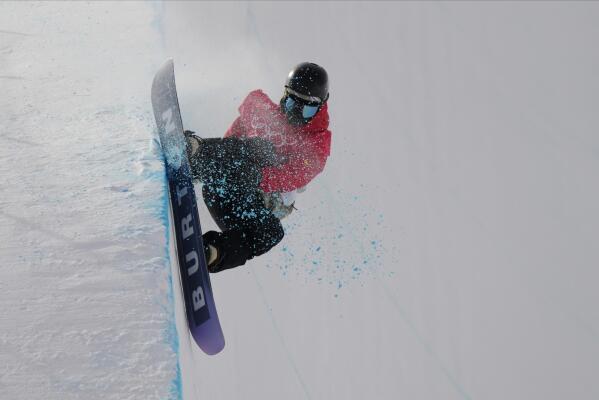The image is an outdoor photograph showcasing a snowboarder skidding to a halt at the edge of a steep, snow-covered drop-off. The snowy landscape surrounding the snowboarder is completely white, with a distinct, thin blue line marking the transition between the flat surface where they've stopped and the steep drop. The snowboarder is dressed in a red jacket adorned with Olympic white rings, black snow pants, a black helmet, and large black goggles. Their snowboard, captured in a vertical position with snow spraying around, is black and purple with the word "Burton" prominently written in white on its bottom. The overall angle of the photograph appears to be tilted, with the snowy wall to the left and the drop-off to the right, enhancing the dramatic effect of the scene.